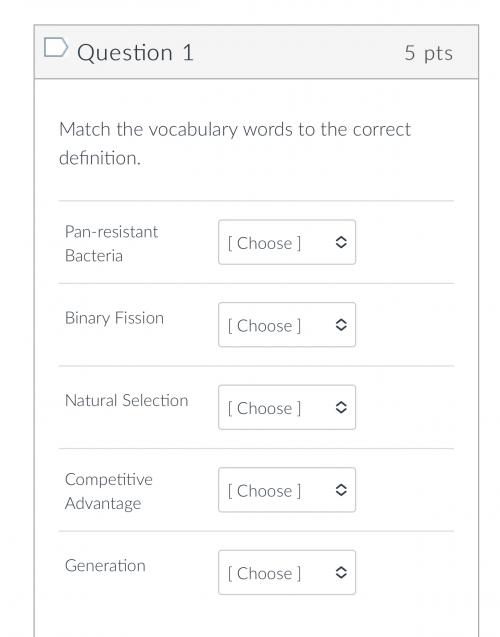The image depicts a light gray header banner with a unique shape that features flat tops and sides, culminating in a pointed center on the right. The banner contains the text "Question 1" with a capitalized 'Q' and the numeral '1,' followed by "5 pts," where 'pts' is an abbreviation for points. Below the banner, on a white background, the question instructs users to "Match the vocabulary words to the correct definition." There are five questions listed, each with a vocabulary term and a corresponding drop-down menu for selecting an answer. The vocabulary terms are: "pan-resistant bacteria," "binary fission," "natural selection," "competitive advantage," and "generation," each accompanied by an up and down arrow for selection purposes.